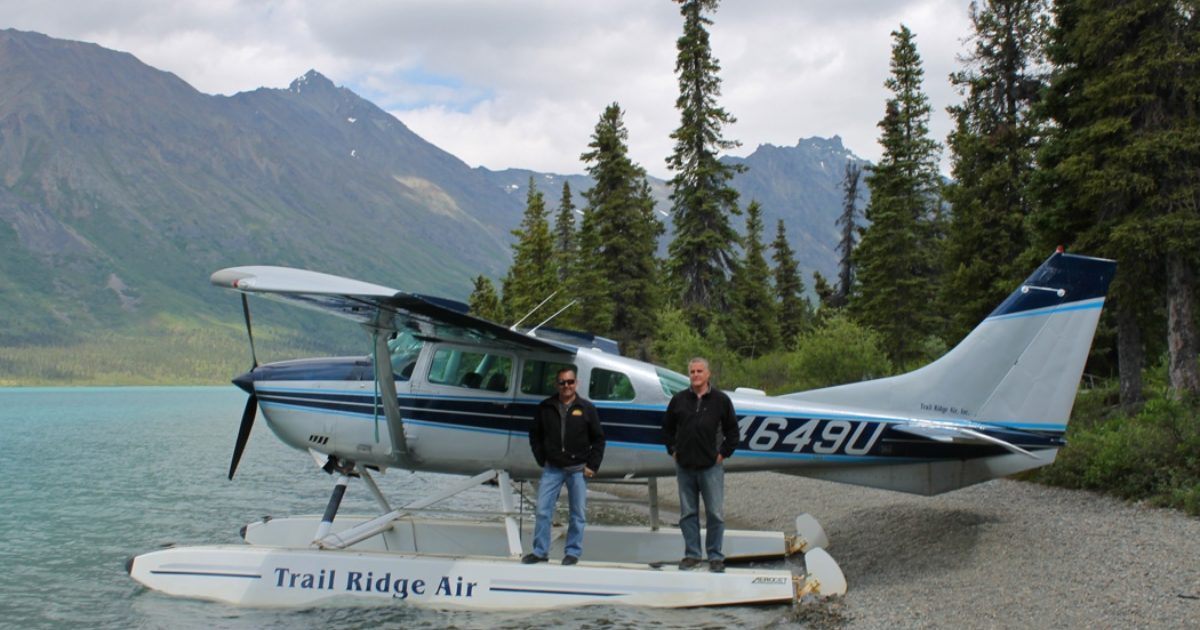In this full-color, horizontally rectangular photograph taken outdoors on a cloudy day, a white and blue pontoon plane labeled "Trail Ridge Air" with "4649U" visible is floating at the water's edge of a lake or beach. Standing on one of its pontoons are two Caucasian men; the one on the left has dark hair and sunglasses, while the one on the right has gray hair. Both are dressed in black jackets and blue jeans. The background features layers of natural elements: a mountain range with hints of snow stretching across the upper left, and lush pine trees and bushes especially prominent to the right and middle. The scene captures a mix of blue, gray, white, green, brown, and silver hues, encapsulating the serene yet dynamic environment under a predominantly cloudy sky.